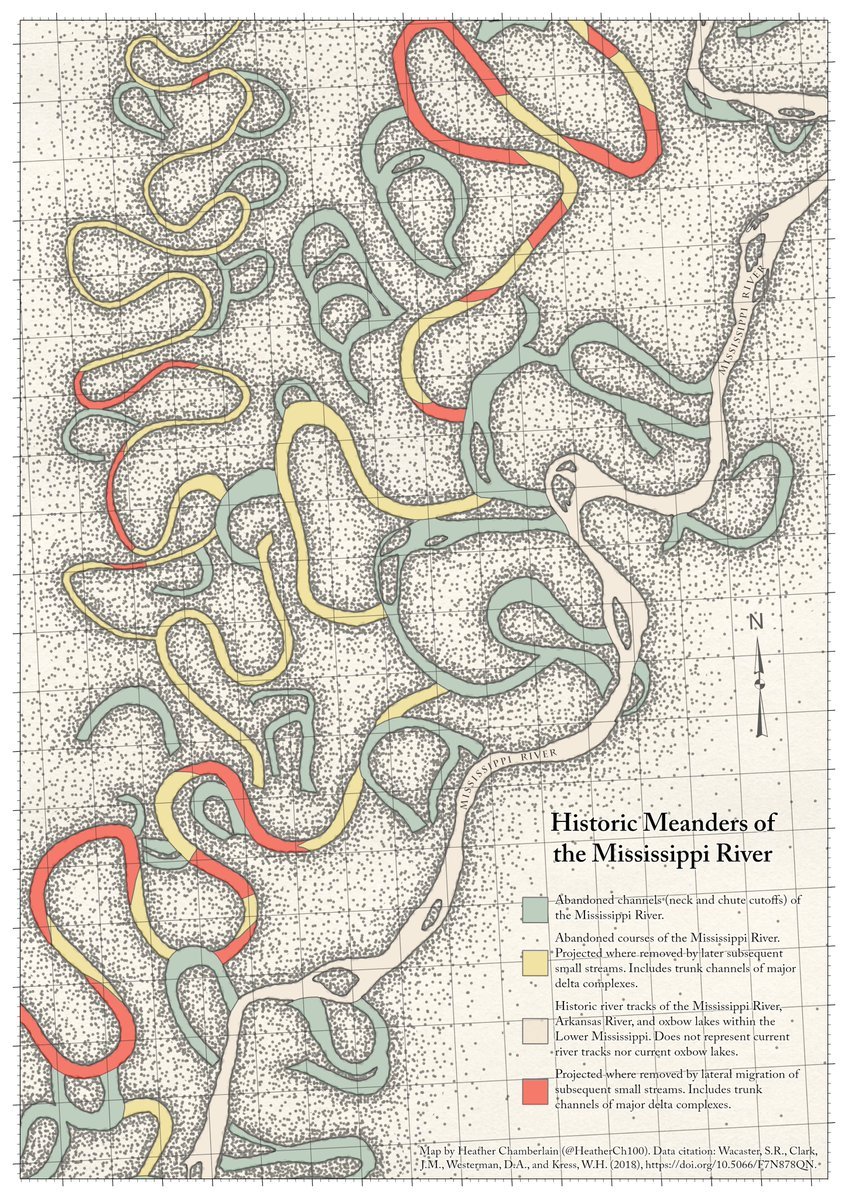The image is a vertical map titled "Historic Meanders of the Mississippi River," displayed in black text. The background is a light beige color with a faint gray grid angled slightly. The map intricately shows various swirling, looping paths of the Mississippi River, represented in multiple colors—green, yellow, red, and white—indicating different historical flow patterns and changes over time.

The green lines denote abandoned channels and neck and chute cutoffs of the river. Yellow lines represent the abandoned courses of the river, affected by subsequent small streams and including trunk channels of major delta complexes. Red lines show areas where the river's courses were removed by lateral migration of smaller streams, also including these trunk channels. The white marks depict the historic tracks of the Mississippi River, Arkansas River, and oxbow lakes within the lower Mississippi Delta, excluding the current river tracks and oxbow lakes.

There are numerous black dots scattered throughout the map, possibly indicating data points or topographical features. Although the black text explaining the different colors is challenging to read, it provides insight into the historical changes of the river's path. The bottom of the map credits Heather Chamberlain as the mapper and cites data from Warcaster SR, Clark JM, Westerman DA, and Kreese WH, 2018, with a partially unreadable URL for the full citation.